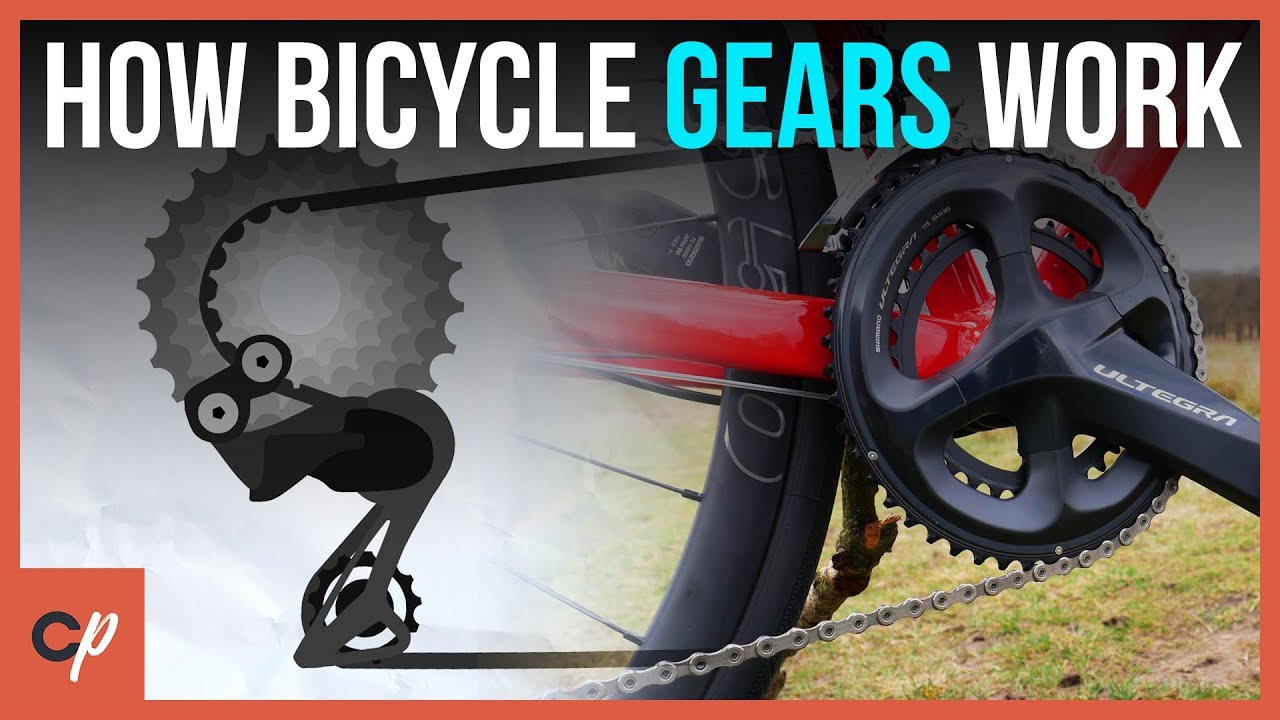This thumbnail, which appears to be an advertisement for an informative video titled "How Bicycle Gears Work," is vibrantly designed with a rectangular shape and a bold orange border. At the top, the title is prominently displayed in large, bold font: "How Bicycle" and "Work" are in white, while "Gears" is in light blue. Below the title, the main image features a red and black bicycle with a silver chain set against an outdoor backdrop of grassy terrain with dirt patches and distant trees under a cloudy sky. To the left of the bicycle, there's an artistic depiction of a bike gear. The bottom left-hand corner carries a square orange logo with the initials "CP," where the "C" is black and the "P" is in white script. The overall composition is clean and visually appealing, effectively highlighting the intricacies of bicycle gears.